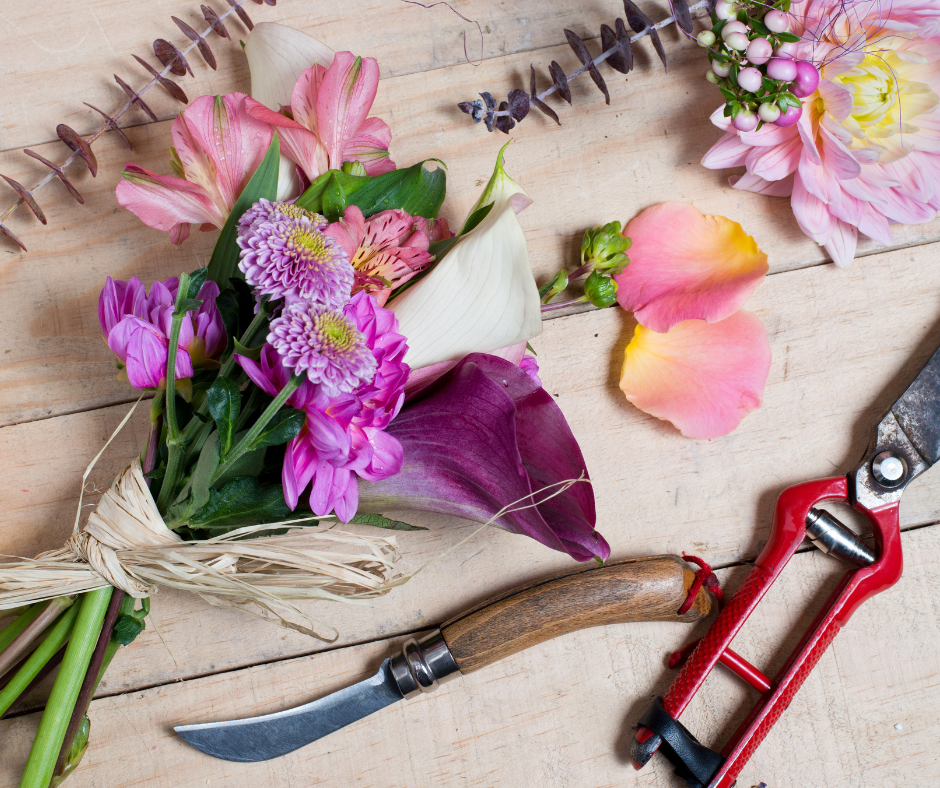In this horizontal rectangular image, a floral arrangement is being crafted on a white wooden tabletop with visible planks. Central to the scene is a bouquet tied with straw or twine, featuring various pink flowers, along with some purple flowers bordered with white, a large white flower, green leaves, and other greenery. Scattered around the table are additional flower petals and loose flowers, predominantly in shades of pink. Tools essential for the arrangement are also visible: a pair of clippers with red handles and a blade extending out of frame, and a curved-blade knife with a wooden handle. In the upper right corner, a large pink flower lies next to smaller pink flowers, while the top of the image shows remnants or cuttings, including long-stemmed items with rounded brown and black petals. The entire setup exudes an atmosphere of artistic floral crafting on a light beige wooden table amidst a backdrop of creative disorder.